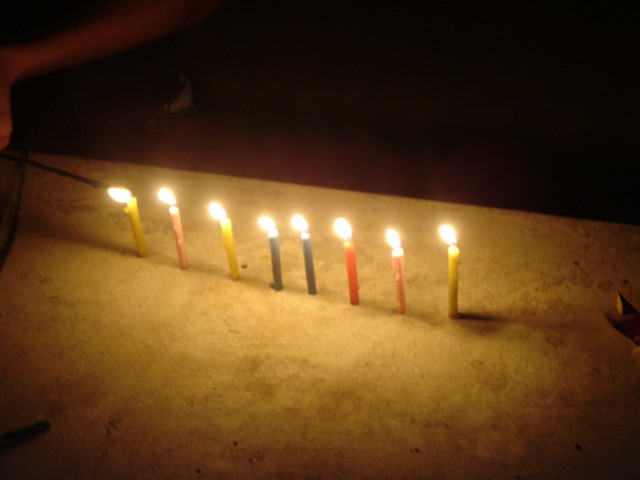In a dimly lit photograph, seemingly taken at night, a row of ten star-shaped birthday candles is planted upright on a concrete slab. The darkness envelops the top portion of the image, where a faint reddish hue can be discerned amidst the blackness. Creeping in from the top right corner is the partial silhouette of someone's arm, holding what appears to be a long black lighter. The lighter is outstretched, lighting a yellow candle on the far left, while the flames of the other candles flicker in a single direction, likely due to the wind.

The candles are arranged meticulously from left to right, featuring an alternating array of colors: yellow, peachy-pink, yellow, two green, red, peachy-pink, and yellow once more. Despite their typical association with birthday cakes, these candles stand solitary on the concrete, unanchored by any holder. The scene evokes a sense of celebration detached from tradition, with the candles' bright hues illuminating the surrounding darkness. The sparse details and shadowy backdrop give the image an enigmatic, almost surreal atmosphere, as if the concrete slab is the stage for a unique, outdoor birthday ritual.